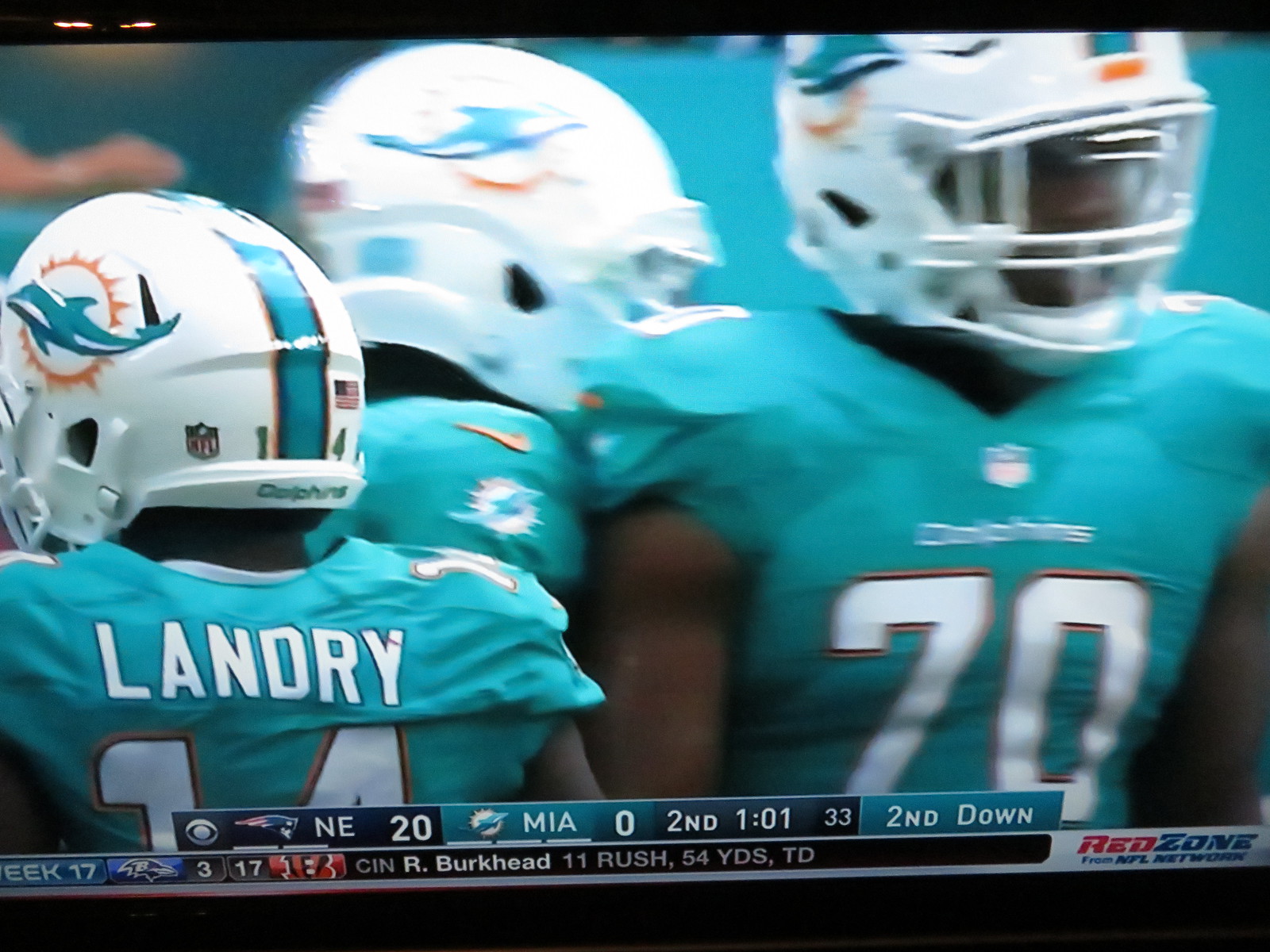This image captures a photograph of a television screen displaying an NFL game between the Miami Dolphins and the New England Patriots. The screen prominently features three Miami Dolphins players. The player with his back to the camera is identified as Landry, wearing jersey number 14. Another player stands to the right of the frame with part of his teal-colored jersey and helmet visible, adorned with a Nike swoosh and the Dolphins logo featuring a dolphin overlaid on a sunburst with orange rays. The third player, partially obscured by the on-screen score bar, appears to be wearing jersey number 70 or possibly 20, though the first digit is cut off. Below the main action, the score insert shows New England leading 20-0 with 1:01 remaining in the second quarter and 33 seconds left on the play clock. It is second down. The lower strip of the screen displays additional NFL information, indicating it's Week 17, and shows a score of Baltimore Ravens 3 to Cincinnati Bengals 17, noting that Cincinnati’s R. Burkhead has 11 rushes for 54 yards and one touchdown. Also visible in the lower right corner is the “Red Zone” logo from the NFL Network, emphasizing that this broadcast compiles scoring plays or critical game moments.